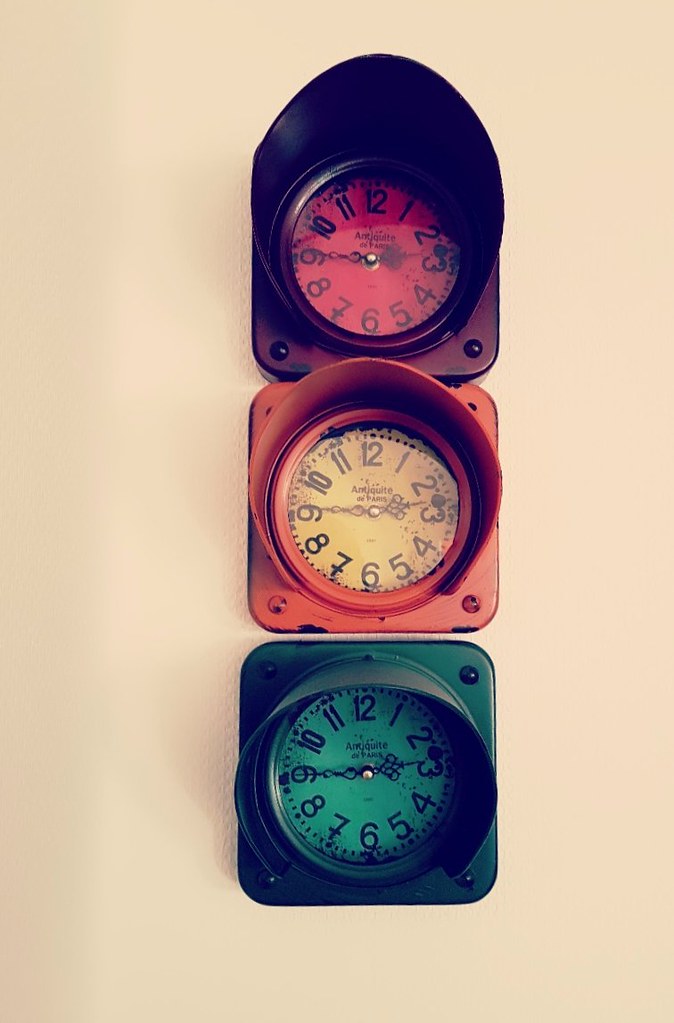The image features a unique clock crafted from repurposed parts of an old stoplight. Each section of the stoplight has been meticulously spray-painted in a dark red, an orangey-yellow, and green. Embedded within each section is an analog clock, all set to 2:45, with identical design save for their color variations. The clock faces are shielded by colored glass that matches each section—red, yellow, and green respectively. These three clocks are mounted on a yellow wall, arranged in a vertical column, effectively replicating the appearance of an actual stoplight.